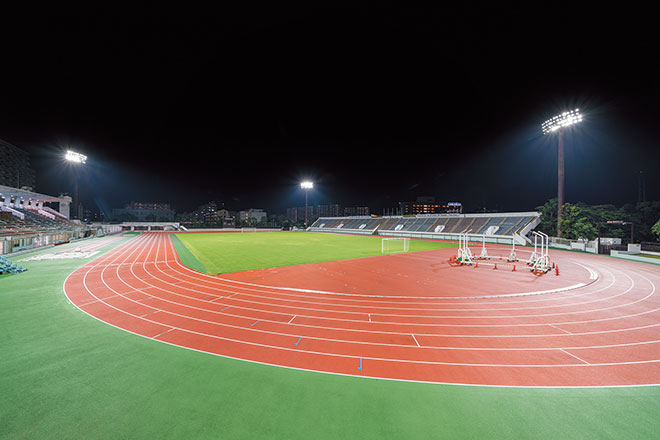This nighttime photo, taken in landscape layout, showcases an athletic stadium featuring a track and a central soccer field. The track itself is an orangey-red color and surrounds a lush green field, marked by two white soccer goals. Encircling the track are multiple white lines demarcating its seven lanes. The stadium is illuminated by three large overhead lights, casting a glow over the scene, and the black night sky dominates the upper half of the image.

On both the left and right sides of the field, metal stadium seating is visible, flanking the track. In the far right, a few trees can be seen, and in the distance beyond the seating, high-rises of six to eight stories tall provide a backdrop. Additional details include orange cones and white hurdles positioned in some areas of the track. The bottom edge of the image features more green areas outside the track, tying together the detailed and orderly layout of this empty, well-lit stadium.